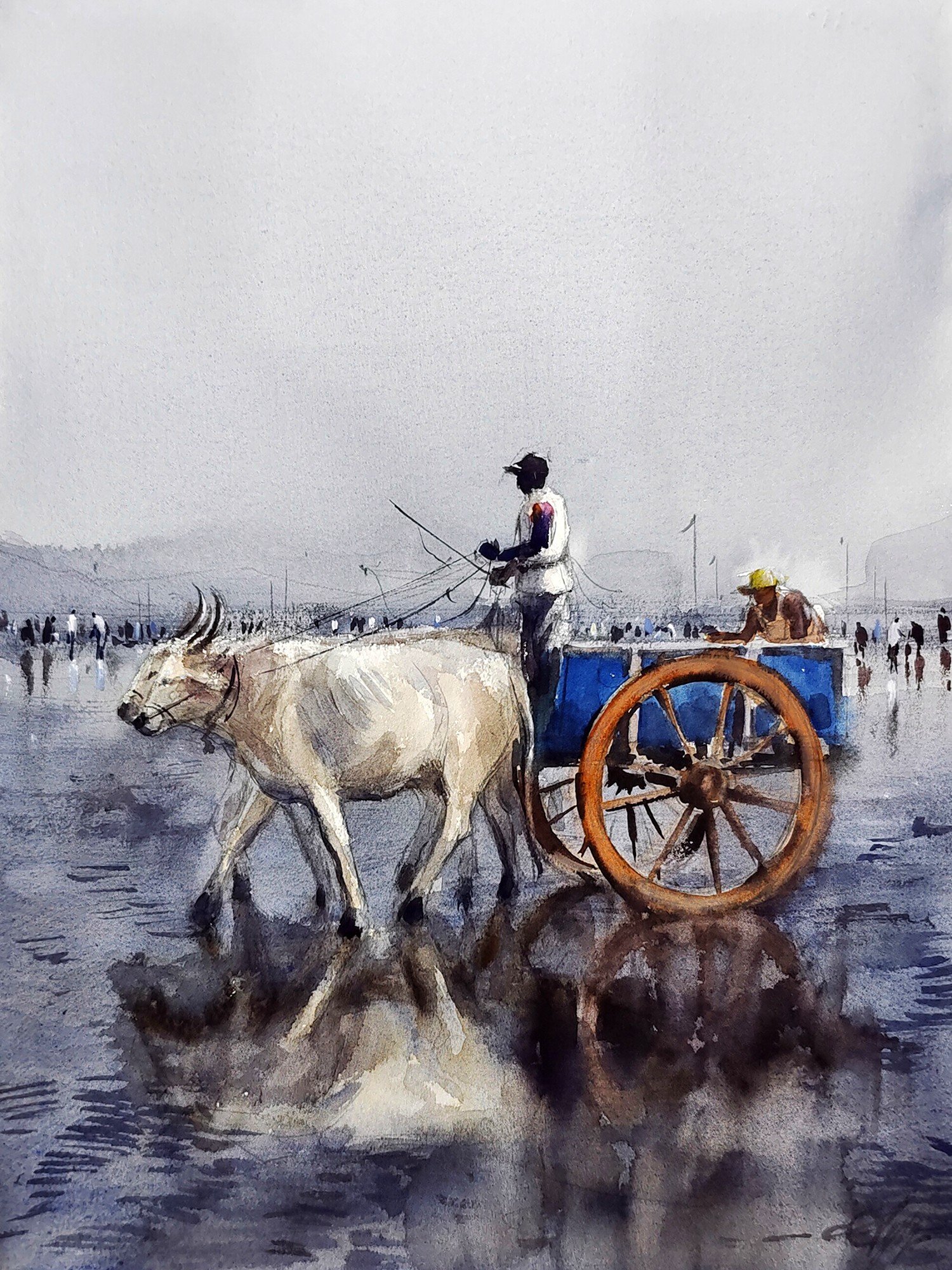This oil painting captures a dynamic scene of a blue cart being pulled by two white oxen with prominent horns. The cart, notable for its large brown wooden wheels, is driven by a man standing up, wielding a switch to guide the oxen through a shallow, reflective water surface. Accompanying the driver is a passenger seated at the rear, distinguishable by a yellow hat. The scene evokes a rural Indian landscape, enhanced by the animals and the attire of the individuals. The background features a misty, grayish atmosphere with mountains barely visible amidst the fog. A crowd of people, depicted in dark, muted tones, populates the distant background. The sky overhead is overcast with wisps of gray clouds, adding to the damp, rainy ambiance. Poles with windsocks stand out whimsically, adding an enigmatic element to the composition.